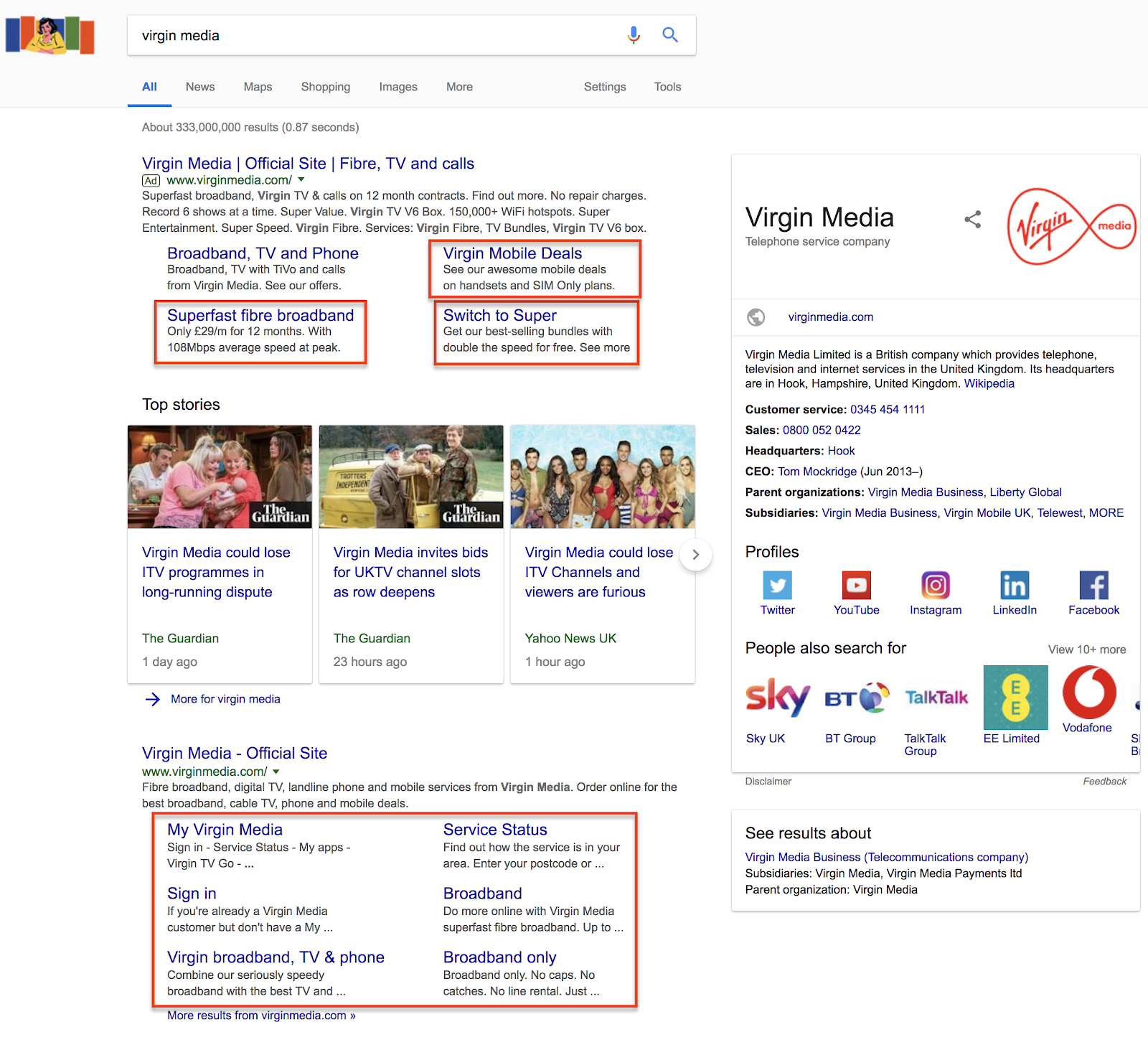This image captures a screenshot of a Google search results page. In the top left corner, a distinctive Google Doodle features a woman with shoulder-length black hair clad in a long-sleeved yellow shirt. She is seated in front of several colorful rectangular objects in dark blue, orange, yellow, and green.

At the center of the page, the iconic Google search bar dominates, its white background contrasting with the black text that reads "Virgin Media." To the right of the search bar, there’s a blue and red microphone icon for voice search and a blue magnifying glass icon for initiating the search.

Below the search bar, various clickable category links allow for filtering the results: "All," "News," "Maps," "Shopping," "Images," and "More." "All" is highlighted in blue and underlined, indicating it is the selected filter. To the right, additional options "Settings" and "Tools" are listed in medium gray.

The search results indicate that there are approximately 333 million results found in 0.87 seconds. The first result listed under "Virgin Media" is prominently displayed, followed by several significant results outlined with a red border, such as "Super Fast Fiber Broadband," "Virgin Mobile Deals," and "Switch to Super," all in blue text.

A "Top Stories" section underlines the importance of recent news, showcasing rectangular thumbnail images of relevant articles with visible human figures.

Further down, another section for Virgin Media includes multiple key options also bordered in red, featuring links like "My Virgin Media," "Sign-In," "Virgin Broadband, TV and Phone," "Service Status," "Broadband," and "Broadband Only," each in blue text.